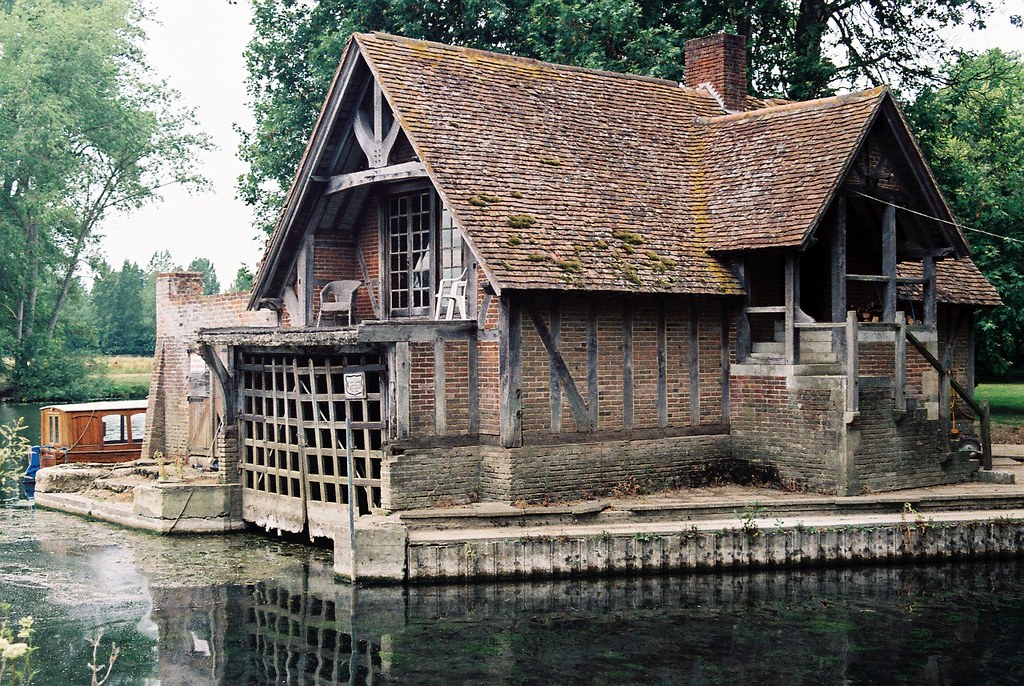The image features a horizontally aligned rectangular photograph of a dilapidated, one-story red brick house with vertical wooden posts embedded between the brick joints. The structure sits precariously on a concrete pier or slab adjacent to a murky, blackish-gray body of water cluttered with debris, including dead leaves, lily pads, and moss. The house boasts a sharply pitched, triangular brown roof covered in light and dark green moss, with a red chimney poking out from one end. 

On the top of the house, there is a small balcony without railings, equipped with two white plastic chairs. Below this, a large wooden gate with a grid pattern appears to open into the water beneath, suggesting access for a boat. Stairs on the right-hand side of the house lead up to the front door. 

In the foreground, there is a stone wall separating the house from the surrounding water, while the background is filled with tall trees bearing green leaves and a cloudy gray sky. Adjacent to the house, a small side porch is supported by dusty, wooden posts. The entire scene is enveloped in an atmosphere of neglect, suggesting the house has been long abandoned.